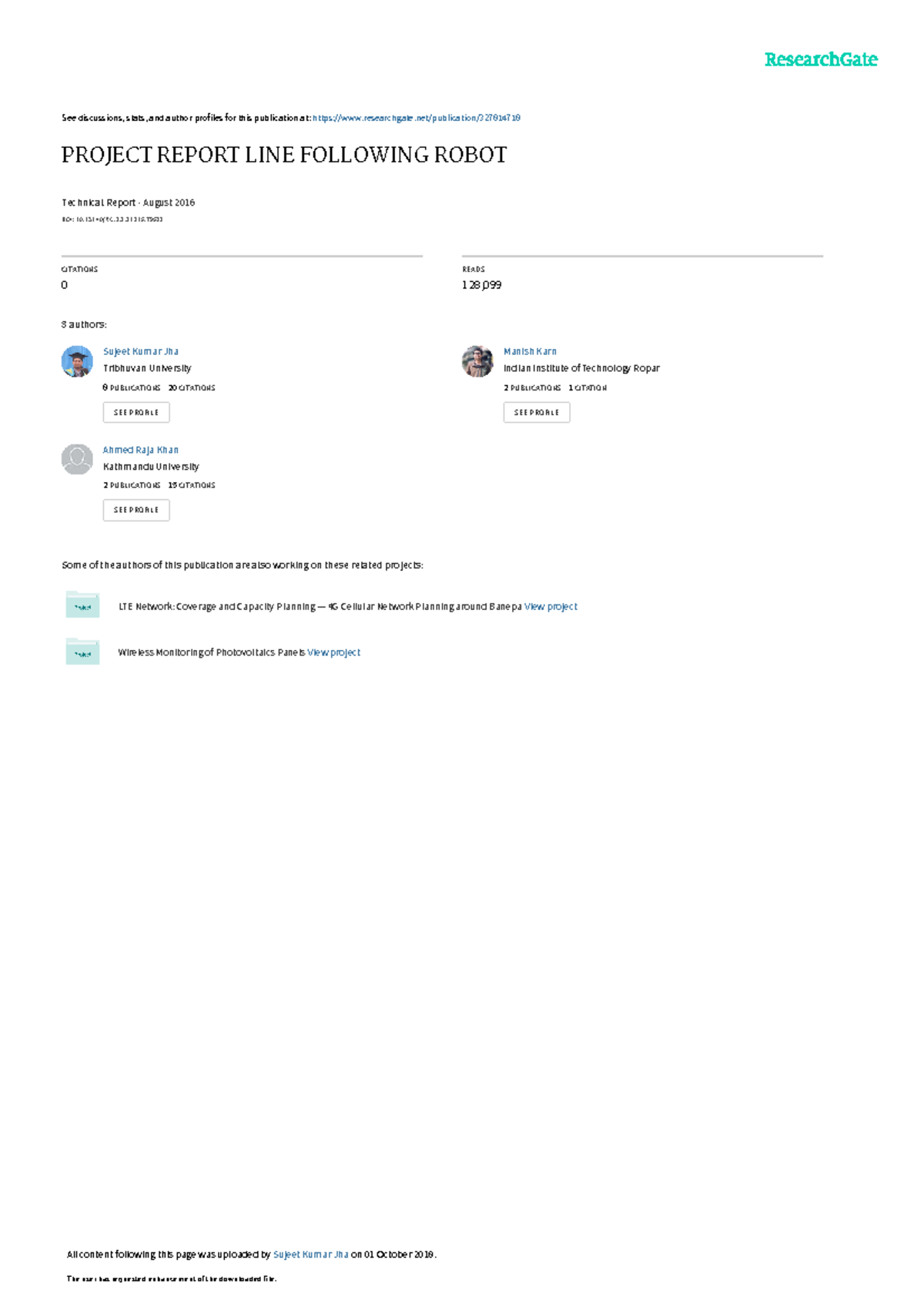The image displays a ResearchGate webpage, which is primarily white, giving it a spacious and minimalist design. The orientation of the image is portrait, approximately one and a half to two times taller than it is wide. At the top, the website banner includes the ResearchGate logo in teal on the upper right corner. Below this, a section of black text and a teal hyperlink are visible but difficult to read due to their small size.

Dominating the upper section of the page, large black capital letters prominently announce the title: "PROJECT REPORT LINE FOLLOWING ROBOT." Directly beneath this line are the author's name and the date of publication, though these details are not legible due to their small font size. Adjacent to or near the author's details, there appear to be two counters—presumably indicating the number of shares or views—with the first counter displaying "0" and the second reading "128,000" and some additional, indistinguishable digits.

Approximately one third down the page, a section headed by the phrase "Three Authors" is visible on the left-hand side, featuring three profile pictures aligned horizontally. Each profile picture has accompanying text, presumably listing the authors' names and affiliations.

Overall, the image provides a structured presentation of an academic project report hosted on ResearchGate, emphasizing the title and authorship while maintaining an airy layout due to significant white space.